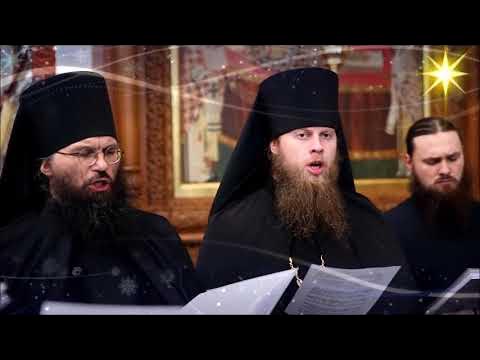In this image, an apparent screenshot from a video, we see three white men participating in what seems to be a religious service. The top and bottom of the image have black borders that indicate it's a screenshot. All three men are dressed in black traditional religious attire. The two on the left are wearing tall black cylindrical hats with veils hanging off the back, and the man in the middle and the leftmost man both have their mouths open, seemingly reciting or singing. 

The leftmost man sports a dark beard, round-frame glasses, and is holding some papers. The man in the center, with a reddish beard, is also holding a piece of paper. The third man, positioned slightly in the background to the right, has dark hair and a beard but no headgear. They all have noticeable beards, contributing to a sense of uniformity in their appearance.

In the background, there's a wall with a large, intricately designed golden-brown framed painting. At the top right corner of the scene, a yellow star is visible. The image features a watermark with spiral designs, further suggesting it might be part of a larger video or broadcast.